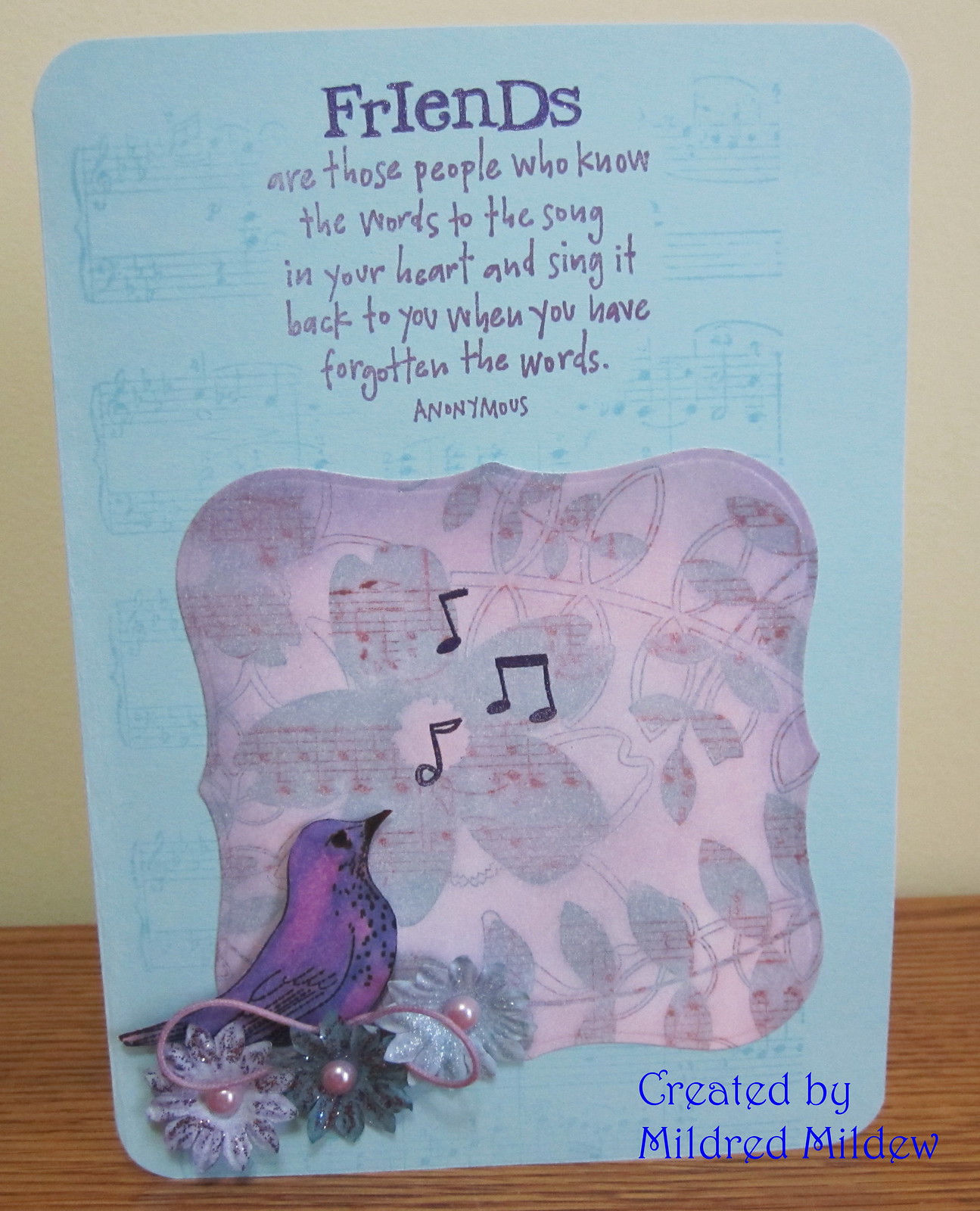The image depicts a rectangular greeting card propped against a white wall on a wooden table. The card, which features a soft blue background adorned with subtle, diluted music notes, prominently showcases a heartfelt quote in whimsical purple text at the top: "Friends are those people who know the words to the song in your heart and sing it back to you when you have forgotten the words." This quote is noted as anonymous. Below this inspirational message is an intricately designed cushion-like motif decorated with muted green flowers and leaves. In the lower left corner of this decorative area, a charming purple bird perches on a trio of sparkly flowers with pearl-like centers. The bottom right corner of the card bears the signature "created by Mildred Mildew," rendered in bright blue. Together, these elements create a visually and emotionally engaging piece that evokes themes of friendship and support.